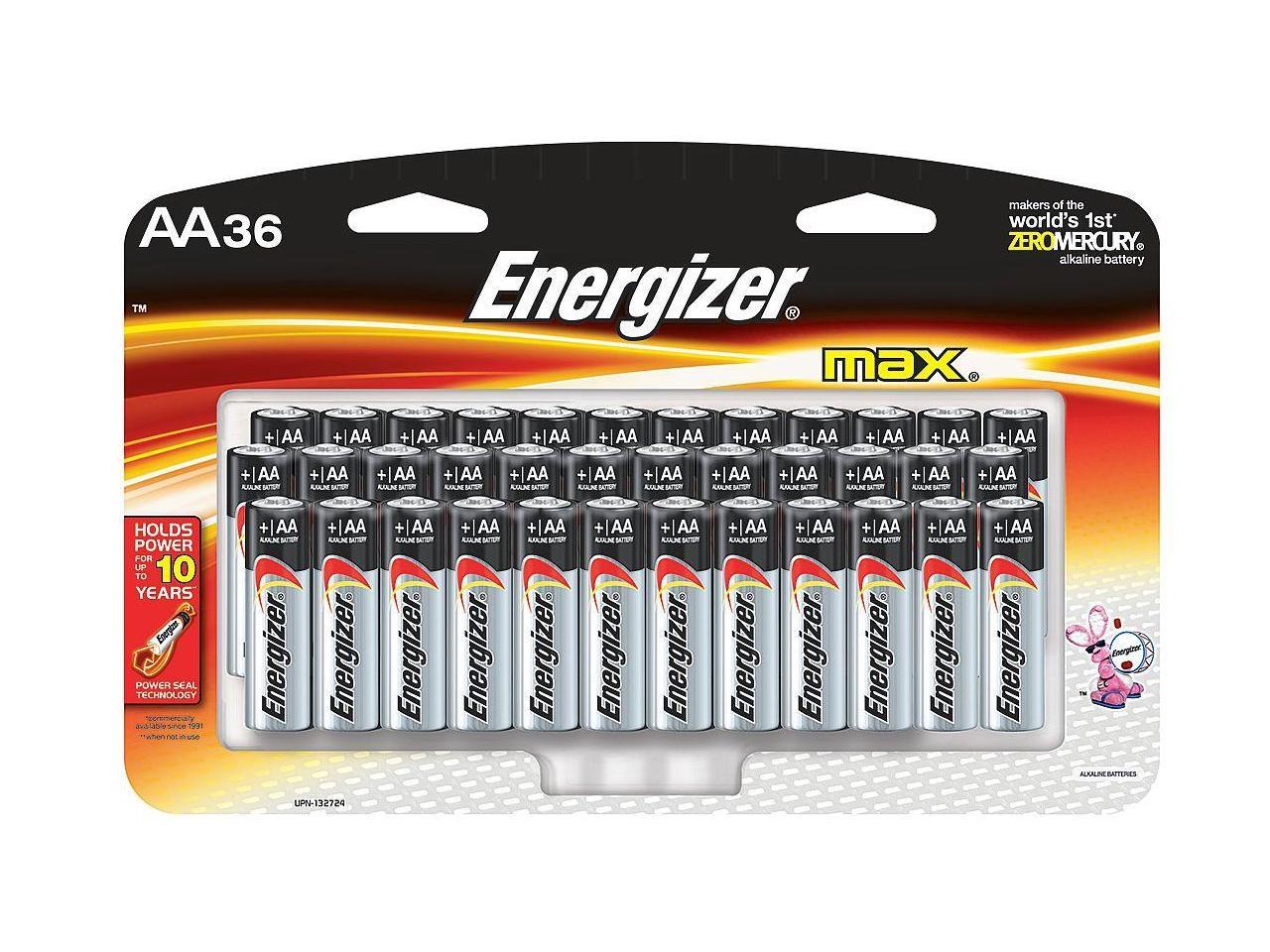Photograph of a blister pack containing 36 Energizer Max AA batteries. The packaging prominently displays the Energizer logo and the claim "makers of the world's first zero-mercury alkaline battery" to the right. At the bottom right, the iconic Energizer bunny is featured banging his drum. Small black text at the very bottom states "alkaline batteries," while the bottom left corner displays the product code UPN-132724.

On the left side of the packaging, it states "holds power for up to 10 years" with an image of a battery and the mention of "power seal technology" below it. Text beneath this is too small to decipher from the photograph. The top left corner reads "AA-36," indicative of the battery size and quantity. The packaging includes triangular cutouts for hanging on wire racks.

The blister pack contains 36 AA batteries arranged in three rows of 12. The packaging is made of a rigid plastic that is often difficult and potentially hazardous to open, a common complaint among consumers.